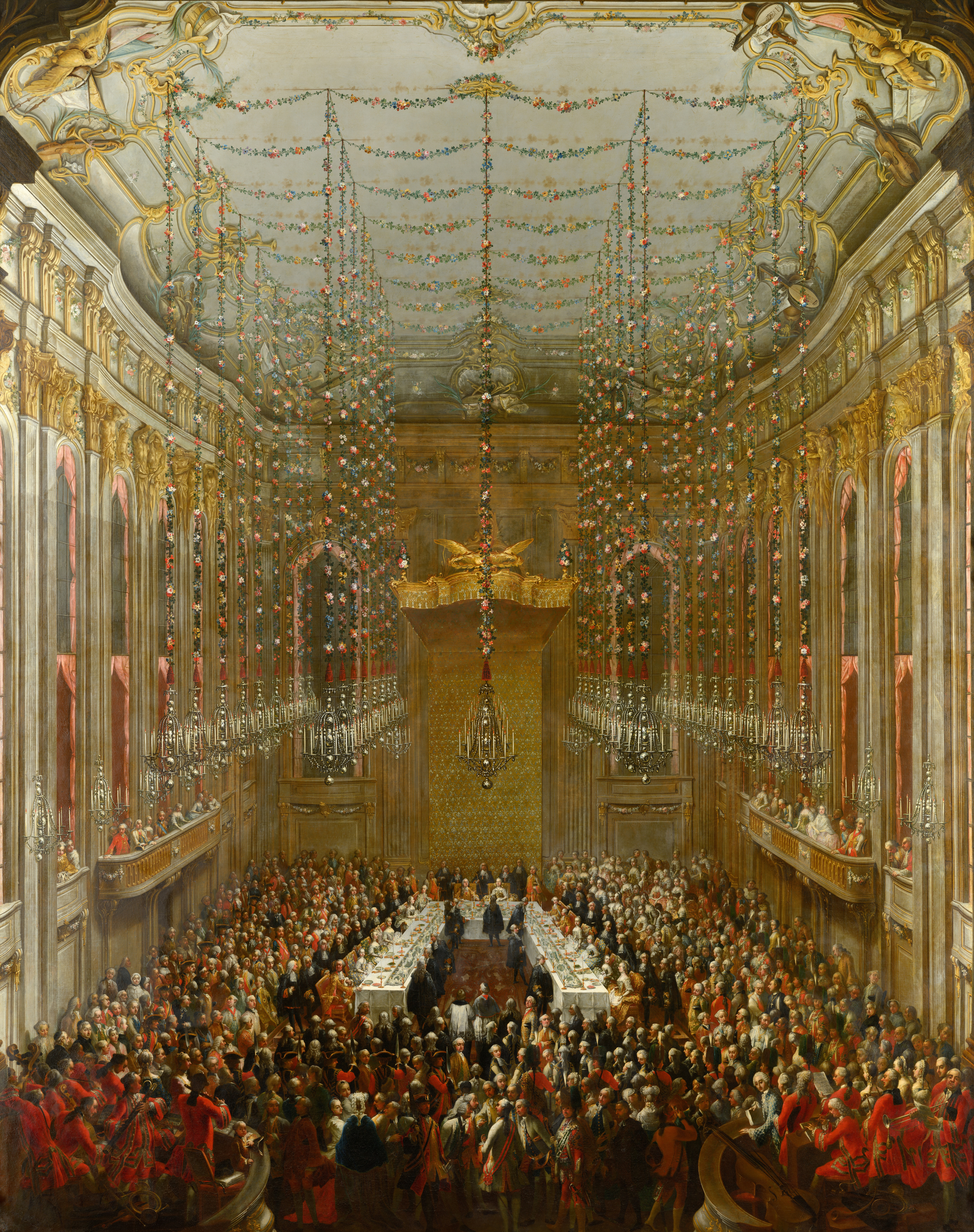The painting depicts an opulent European dining hall, possibly of British or U.S. origin, characterized by its grandiose architecture and luxurious ambiance. The room boasts towering ceilings adorned with multiple chandeliers, reflecting the extravagant décor and high social standing of its occupants. The space is densely populated with elegantly dressed individuals, suggesting a lavish social gathering or banquet.

Two orchestral sections are seen on either side of the hall, providing entertainment to the crowd. At the center of the room, a U-shaped dining table with sharp corners is arranged, surrounded by a throng of guests. Several people are seated at the table, being attended to by waiters who move deftly within the enclosed area of the table's interior. The painting captures the hustle and bustle of the event, highlighting the sheer number of attendees that practically fill the room to capacity. Dominating the entrance to this magnificent hall is an impressive golden door, adding to the overall grandeur and regal atmosphere of the scene.